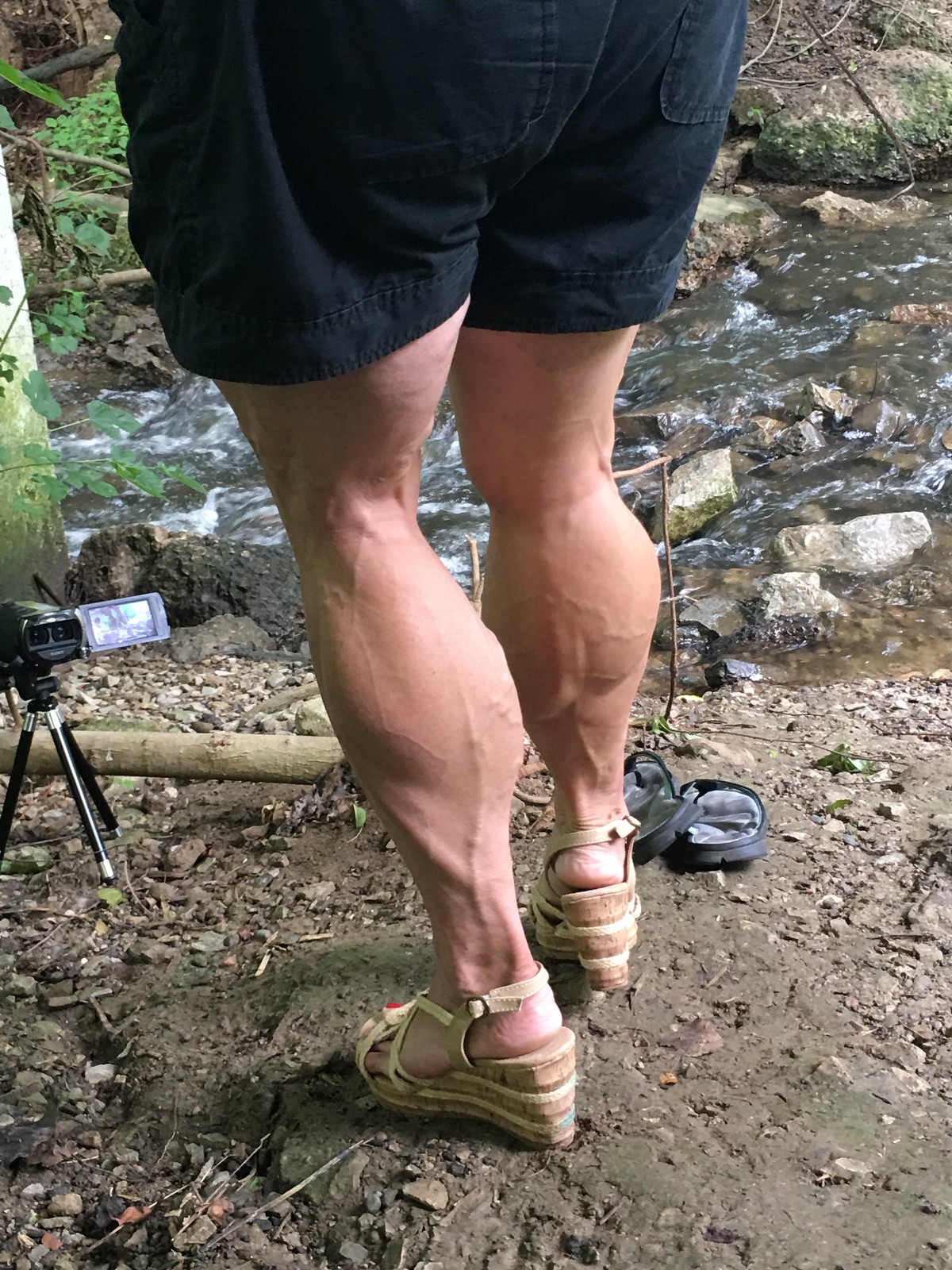The image depicts a muscular older woman standing at the rocky edge of a creek bed, partially concealed by her black shorts which extend less than four inches down her thighs. The bottom half of her body is in view, revealing her extremely well-defined, veiny calves and thighs, suggestive of a bodybuilder. She is wearing tan, open-toed wedge platform sandals with straps around her ankles, and her toenails are painted red. In front of her, close to the ground, is a small black handheld video camera mounted on a mini tripod, its screen facing outward. The camera appears to be set up to film her powerful legs. Surrounding her are the natural elements of the creek bed, including rocks and dirt.